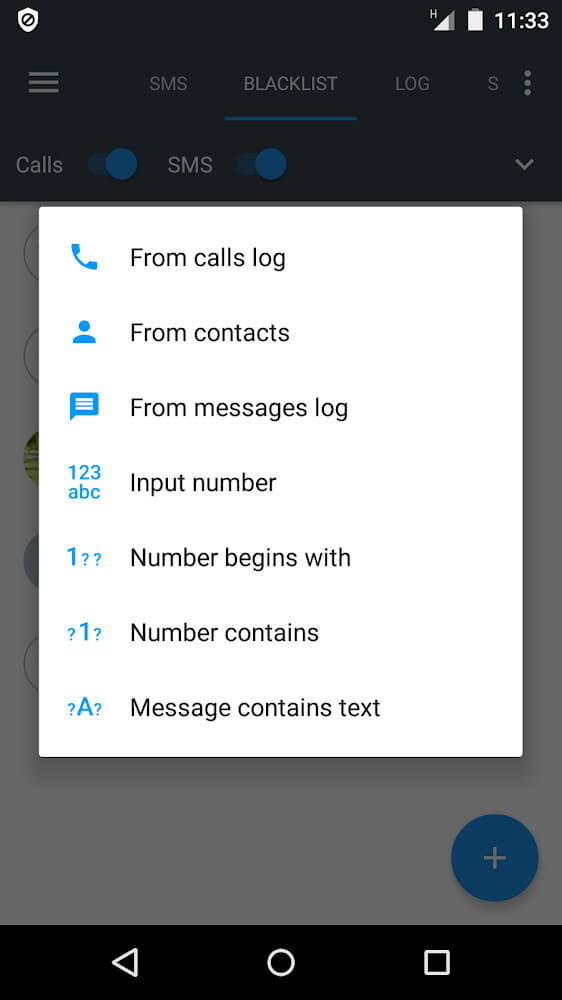The image features a website interface on a mobile device. At the top, there's a black banner with a slightly faded background. On the left side of this banner is a small shield icon, while on the right side, there are icons displaying battery life, cell phone signal, and the current time, "11:33." Below the banner, three horizontal lines are stacked on top of each other, representing a menu button. 

Further down, there are three main headings in capital letters: "SMS," "BLACKLIST," and "LOG." Just beneath these headings, the word "Calls" is displayed, followed by a blue circle icon. Adjacent to this, "SMS" is written again, followed by another blue circle and a dropdown arrow.

At the center of the interface, there's a white pop-up window with various options, each starting with a capital letter. The options listed are as follows: "Call," "From Call Logs," "From Contacts," "From Messages Log," "Input Number," "Number Begins With," "Number Contains," and "Message Contains Text." Each option is accompanied by a small icon. 

At the bottom right corner of the interface, there's a prominent blue circle featuring a white plus sign (+) in the center.